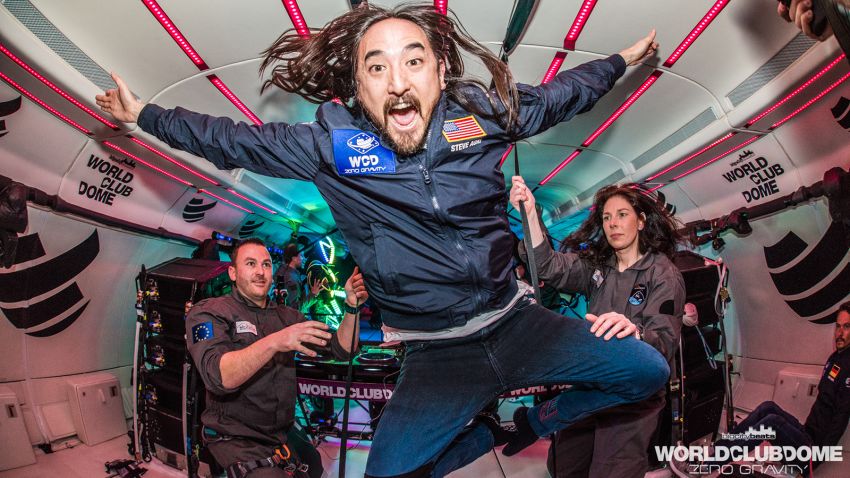The image captures a vibrant scene inside an aircraft-like structure, emblazoned with the words "World Club Dome" and "Zero Gravity" on its sides and bottom. Central to the image is renowned EDM producer Steve Aoki, identifiable by the name on his navy blue jacket adorned with an American flag and a WCD Zero Gravity badge. Aoki, with his long brown hair floating wildly due to the zero gravity environment, has a euphoric expression, arms outstretched and legs bent as if leaping or floating. He wears blue pants, a white undershirt, and black socks, fully embracing the weightless experience.

Behind Aoki, two individuals in grayish or brownish outfits, with blue and black badges, appear to be holding onto something, perhaps stabilizing themselves or participating in the zero gravity setup. The woman among them has long dark hair. The interior of the aircraft features pink LED strip lighting on the ceiling, adding to the festive atmosphere, along with a DJ mixing booth and speakers, suggesting a dance party. The backdrop and setup resemble a DJ booth or disco, emphasizing the image's energetic, celebratory vibe as part of the World Club Dome Zero Gravity experience.